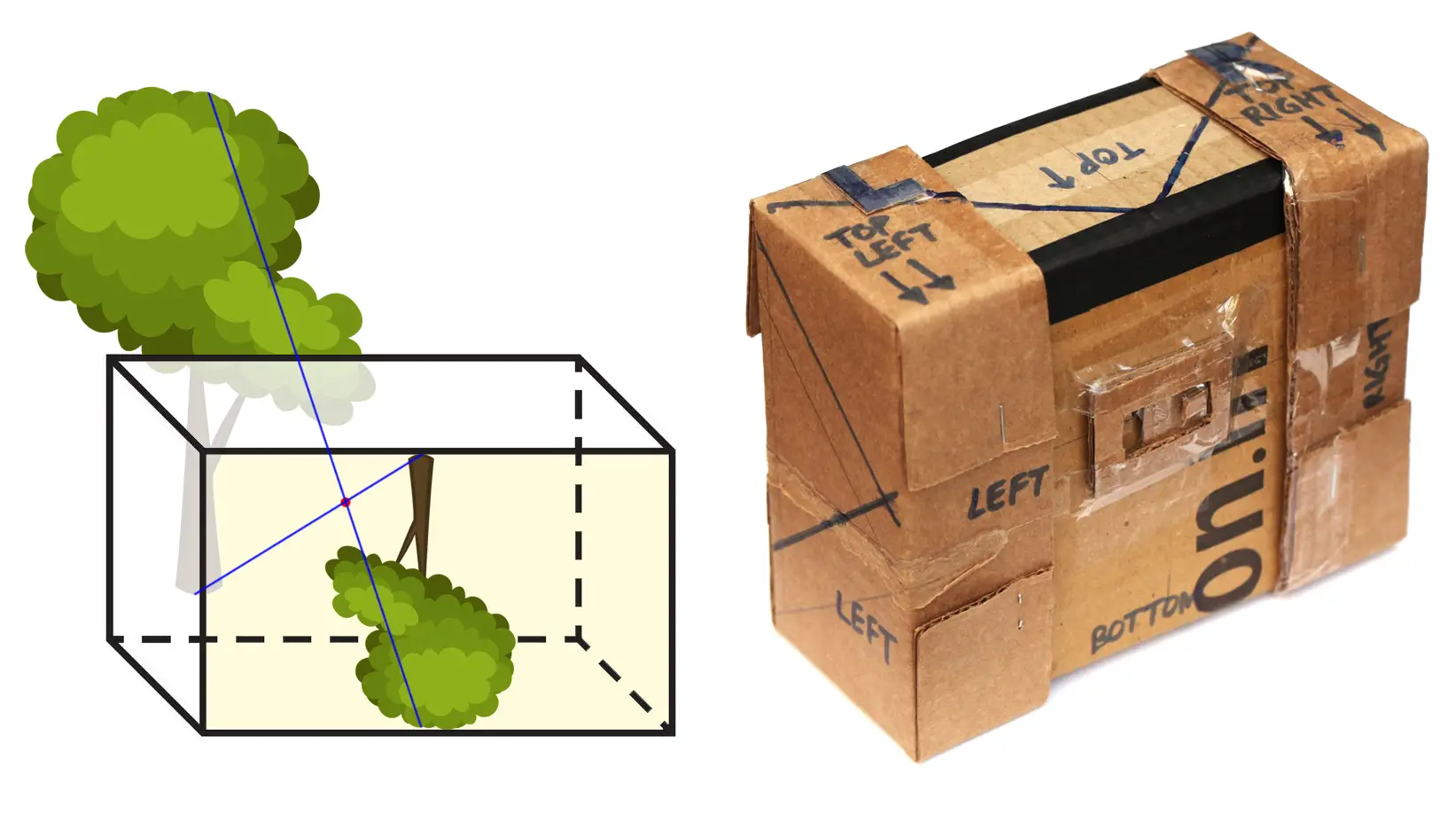The image features a white background with two distinct sections: on the left, a hand-drawn 3D box and, on the right, a photograph of a cardboard box. The left section showcases a 3D rendering of a rectangular box with a clear black outline, detailed with lines and dotted lines to suggest depth. The front panel of this 3D box includes a yellow section displaying an upside-down reflection of a tree, which also appears behind the box with a brown trunk and vibrant green foliage. A blue line runs from the top of the tree inside the box down to the left, exiting the box's bottom. 

On the right, there's a real cardboard box depicted at an angle, showing its left side and front. This box is heavily taped and labeled with various markings: the front bears the notation "ON dot something," while the left side and front corner are marked "left" in black. Additionally, the top-left corner features a large black "L" and the label "top left" with two arrows. The top edge has "top" written upside down with an arrow, and the right side includes an "R" with "right" below it and two corresponding arrows. The front of the box also has a small block of wood taped with the number six, adding another layer of detail to the scene.